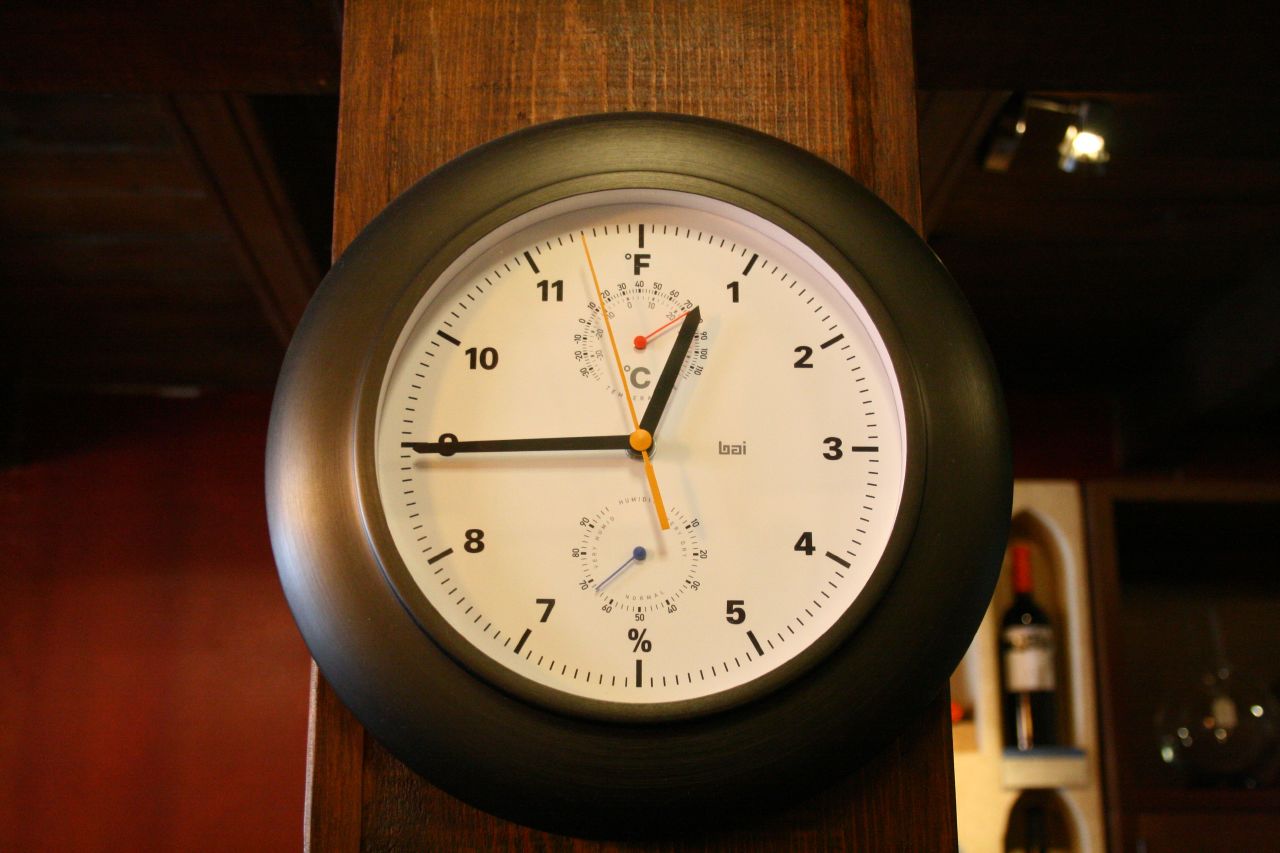The image captures a round analog clock mounted on a vertical wooden beam inside a room, likely a restaurant or wine storage area. The clock features a unique display where traditional numbers are replaced with a mix of characters and numbers: instead of the 12, there's "F°," and instead of the 6, there's a "%" sign. The numbers 1 through 5 and 7 through 11 are present in their usual positions. The clock's white face contrasts with its thick black edges, and it has black hour and minute hands, along with a yellow second hand. Smaller clock drawings are embedded inside the main clock, positioned near the "F°" at the top and the "%" sign at the bottom, both mirroring the main clock's time of 12:45. The scene also reveals part of the room, showing a wall with a white shelf at the bottom right, holding a wine bottle with a red cap, a black base, and a white label, adding to the ambiance of the setting. The overall decor appears wooden, enhancing the rustic elegance of the space.